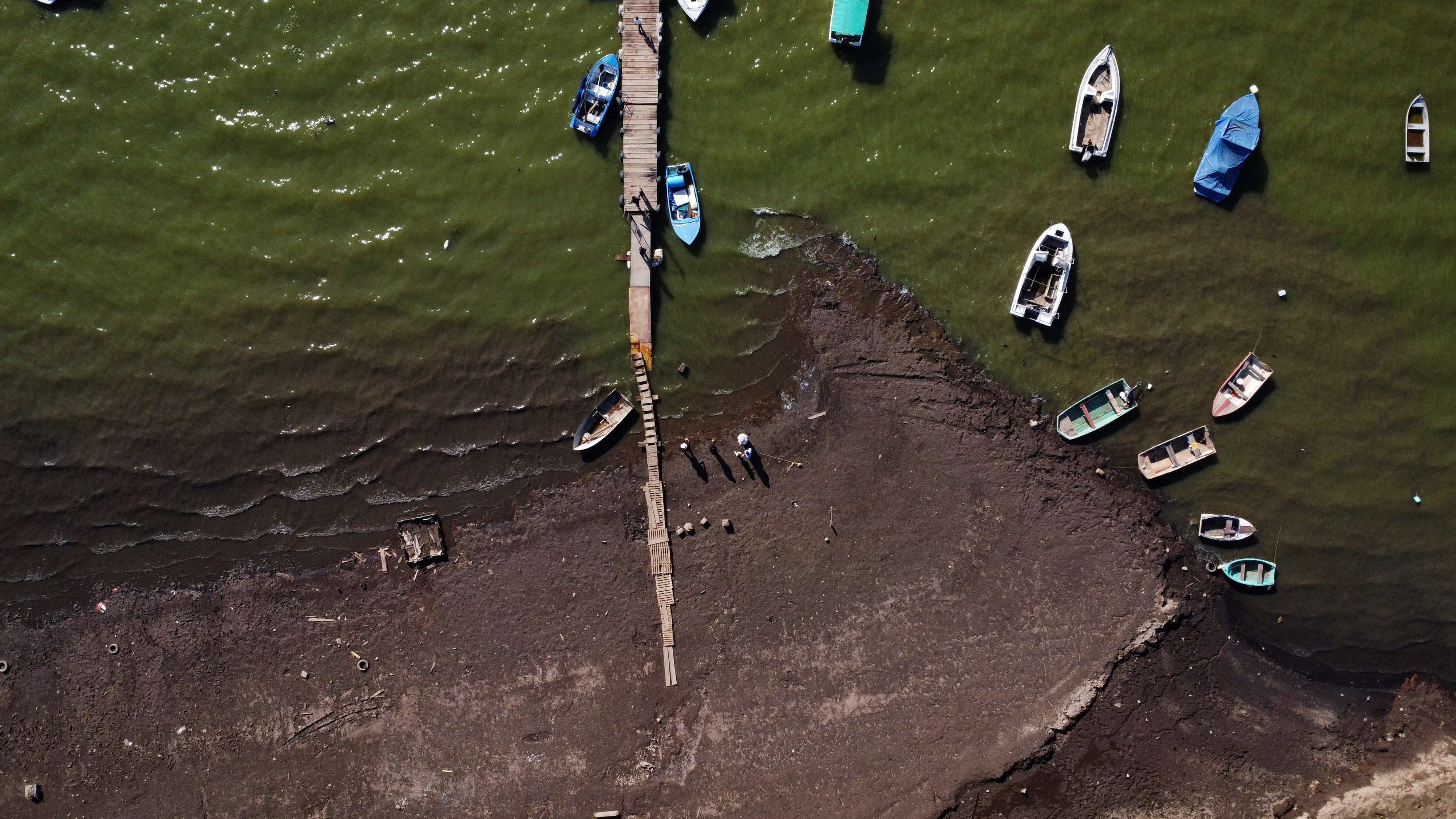A realistic, top-down color photograph captured from a drone showcases a coastal scene viewed from a great height. The brown soil land at the bottom transitions into a basalt-colored beach with several human figures standing and moving about. Extending from the shore is a narrow wooden pier or boardwalk, stretching into the green, murky waters. The area appears to bustle with activity, possibly involving surveyors or locals testing water quality. On either side of this pier, around 12 fishing boats of various shapes and sizes float, primarily small vessels that could accommodate up to three to four people. These boats, some white and some blue, are scattered throughout the water, with about ten on the right side and a few on the left. The setting suggests a collection of fishermen’s boats, possibly in an African or Caribbean locale. An artist’s mark or an object is visible in the lower left corner of the image, adding a subtle point of interest to the composition.